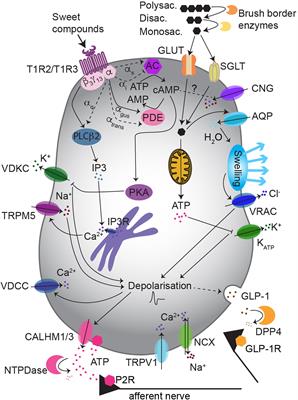This educational scientific diagram illustrates the complex mechanisms involved in the processing of sweet compounds. The central focus is a large white oval, which serves as the substrate displaying various labeled components integral to the process. 

At the top of the diagram, there is a heading labeled "Sweet Compounds" in black text, with an arrow directing attention to a small, devil-head-shaped icon. Adjacent to this, various saccharides are listed, including "Polysaccharides," "Disaccharides," and "Monosaccharides," along with the term "Brush Border Enzymes." These labels are connected to small yellow ovals by black arrows, suggesting a stepwise breakdown or interaction with these saccharides.

On the right side of the white oval, blue circular structures are labeled with abbreviations such as "CNG" (Cyclic Nucleotide-Gated channels) and "AQP" (Aquaporins), indicating the involvement of these channels in the process. Black arrows extend from these labels, pointing to specific sites on the white oval, further highlighting their role in the diagram’s context.

Overall, the image serves as an intricate map of how various components and enzymes interact with sweet compounds, emphasizing the roles of polysaccharides, disaccharides, monosaccharides, and other molecular entities in what appears to be a detailed cellular or biochemical process.